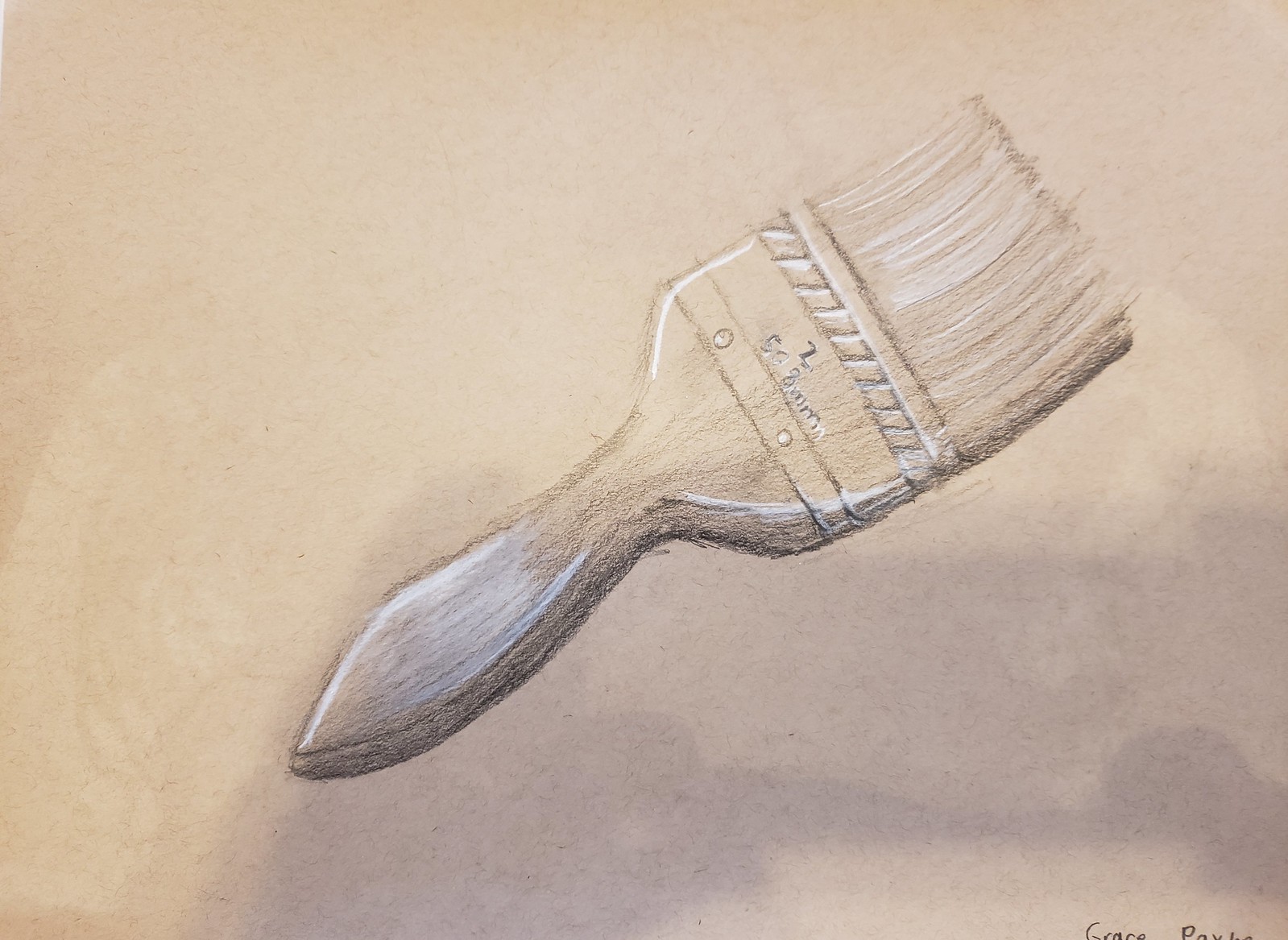The image is a detailed watercolor painting of a paintbrush, positioned on a cream-colored background that varies in intensity, creating a sense of depth with shadows and shading. The focal point is a wide, flat paintbrush angled with its bristles pointing toward the upper right corner of the image, while the handle points toward the bottom left. The paintbrush features a brown wooden handle that is slightly tapered, and the metal ferrule connecting the bristles to the handle is marked with the number "2" and "5028mm." There are two small, wide circles on the metal piece, indicative of screws. The artist's signature, partially visible in the bottom right corner, reads "Grace Pave..." but the complete last name is obscured due to cropping. A subtle beige splotch stretches across the bottom of the image from left to right, adding to the overall texture and depth of the painting.